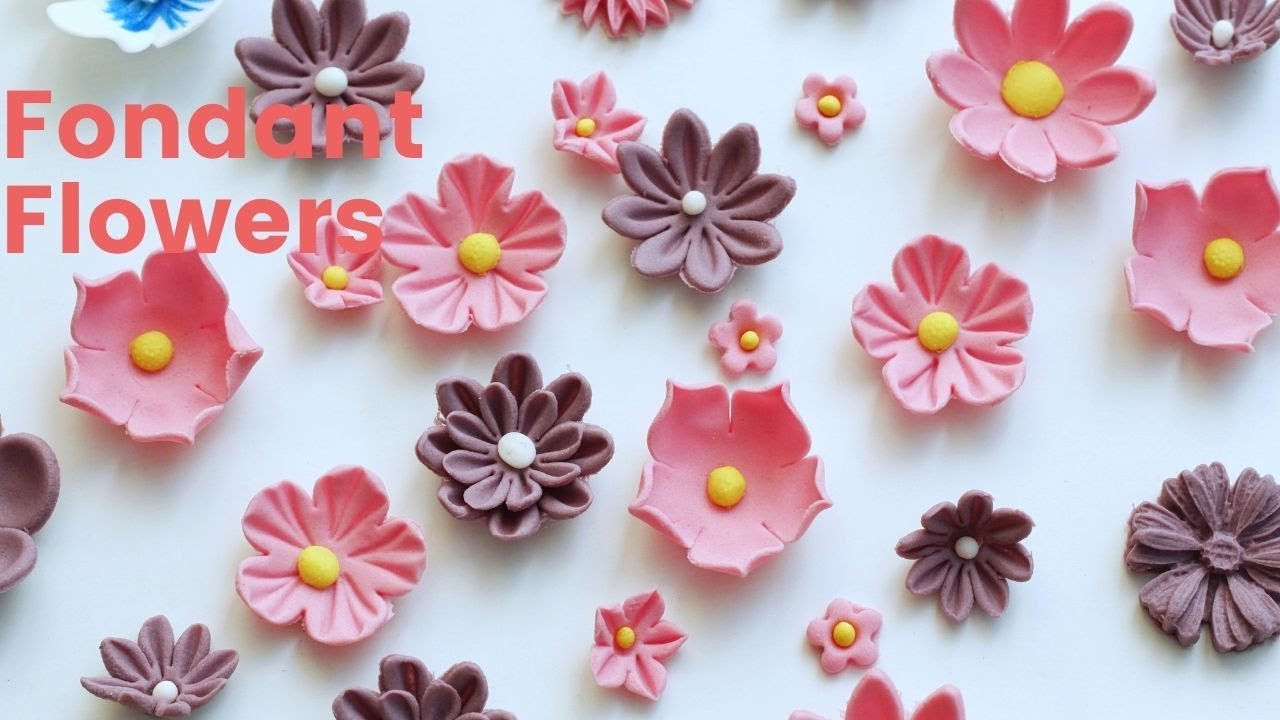This photograph, taken indoors, captures an array of fondant flowers displayed on a white surface, likely a table or board. The image is rectangular, approximately six inches wide by three inches high, and is presented in a landscape format. In the upper left-hand corner, there is pink text stating "Fondant Flowers." The flowers themselves range widely in size, color, and design. Predominantly, there are pink flowers with tiny yellow centers, varying from very small to large. Additionally, there are brownish-purple flowers, most of which feature small white dots at their centers. The pink flowers resemble daisies and some have five rounded petals, while others have upward-curving, pointed petals. The brownish-purple flowers frequently have around six to eight petals, with some even having smaller flowers nestled inside. A notable feature in the upper left corner, just above the text, appears to be either another fondant creation or a bowl, characterized by white rims and a dark blue center.